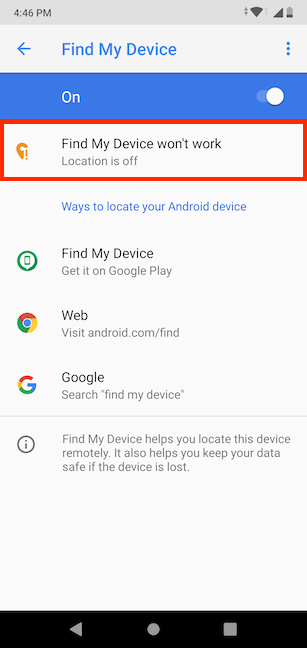A screenshot taken from a smartphone at 4:46 PM shows the user connected to Wi-Fi. The main feature highlighted is the "Find My Device" function, which is currently switched on, indicated by a blue bar. The screen details various ways to locate the Android device, promoting the "Find My Device" app available on Google Play. The app's icon is displayed alongside a message that it aids in locating the device remotely and securing data if the device is lost. The battery is completely depleted, shown by a fully discharged battery icon. At the bottom, a black navigation bar indicates options to return to the home screen. A suggestion to visit android.com is also present.